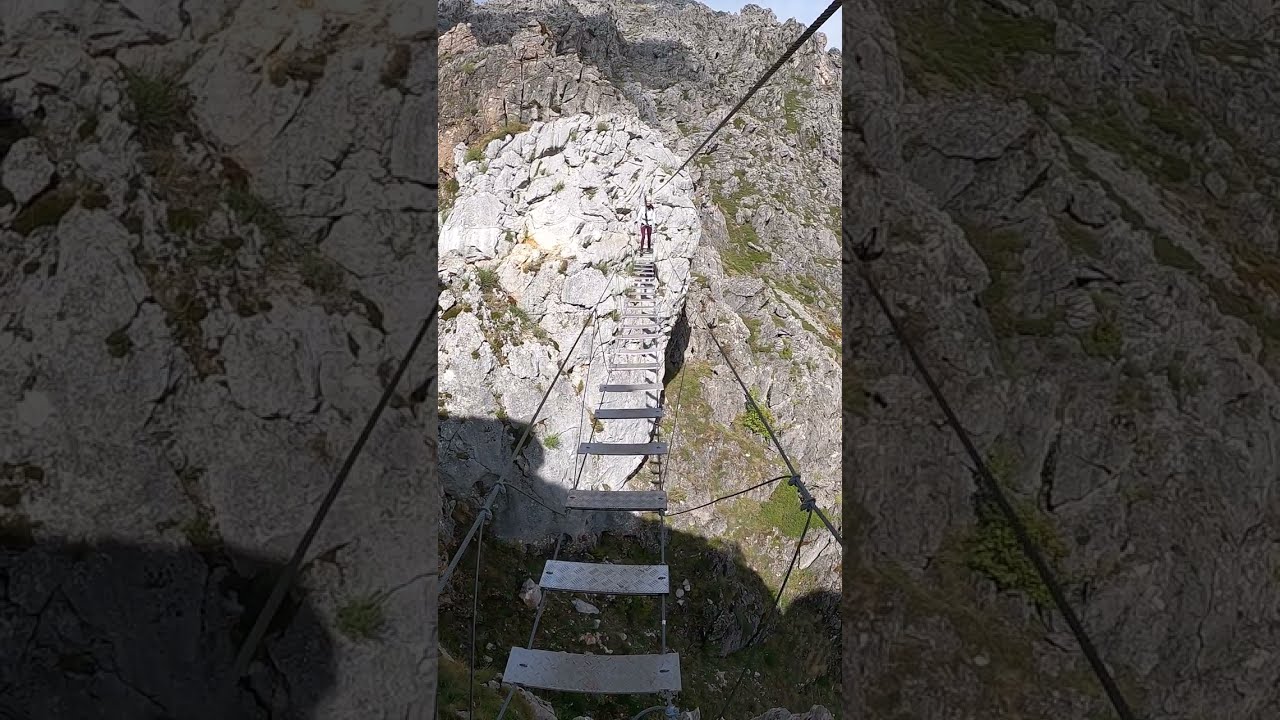The image depicts a striking but precarious hanging bridge spanning between two mountainous cliffs. The bridge structure is supported by sturdy wires and features a floor composed of numerous rectangular silver metal plates, interspersed with open gaps. The surrounding environment is rugged, with an abundance of irregularly shaped stones and rocks. A woman wearing a white helmet, a white long-sleeve top, and purple leggings is seen walking cautiously across the bridge. She is secured with a safety rope, adding a layer of protection against the steep and rocky terrain below. The path ahead appears daunting, as the bridge's steps resemble a high ladder with considerable gaps. In the background, the large, craggy mountain continues to dominate the scene, decorated with patches of green moss and scattered plants. The vivid colors of gray, brown, green, silver, black, white, and blue contribute to the dramatic and natural beauty of this outdoor mountain setting, with a glimpse of the sky visible in the top right corner.